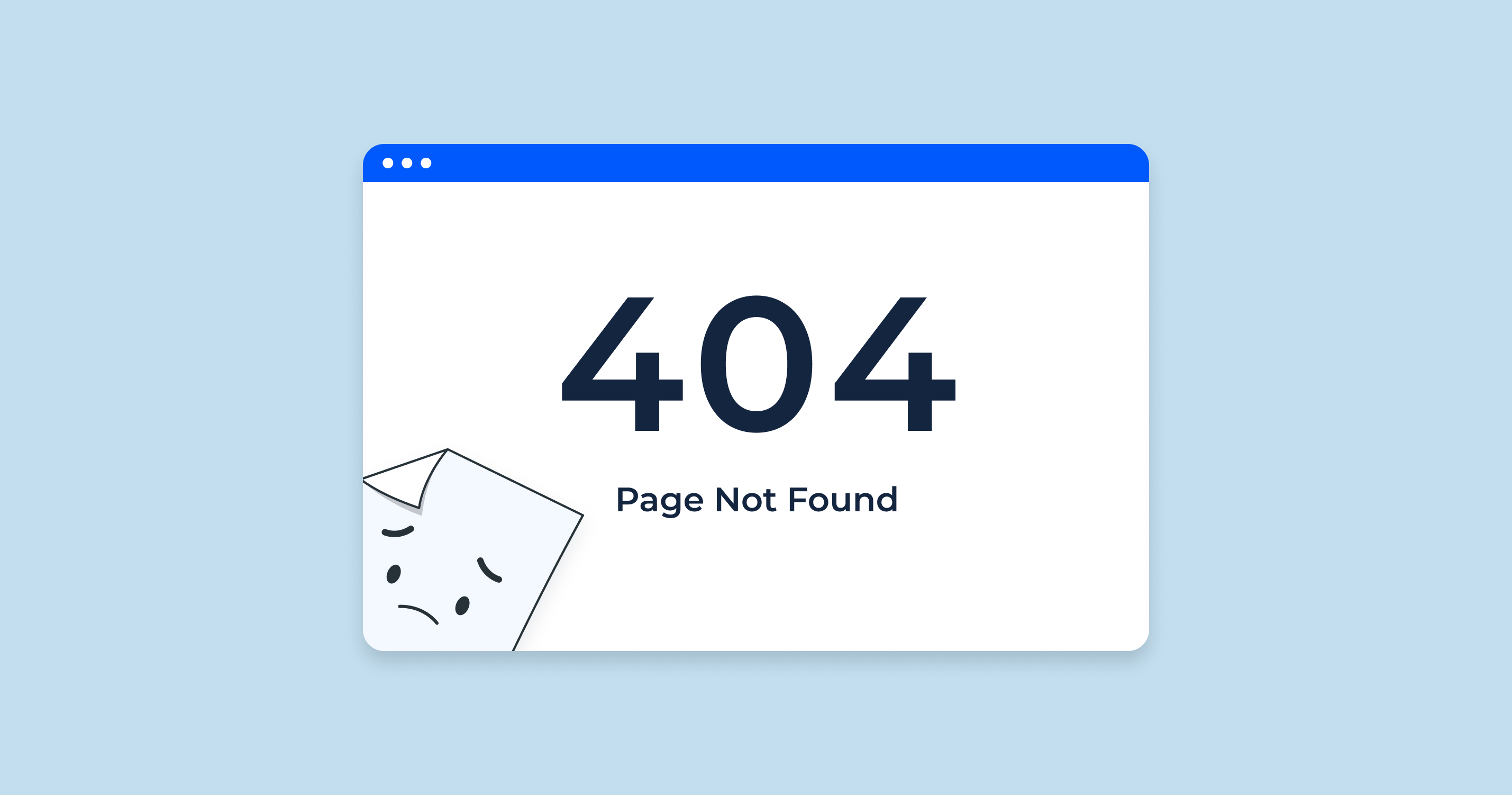The image depicts a "Page Not Found" graphic commonly seen on non-working websites. The background is a pale blue, setting a calm tone. Central to the image is a white text box bordered at the top by a blue line, highlighted with three white dots, which likely indicate more options. Dominating the center of the text box, the number "404" is displayed prominently in a bold font, directly above the smaller text "page not found," both written in black. In the lower left corner of the text box resides a cartoon-like icon of a piece of paper symbolizing the missing page. This icon features a folded top corner and a sad face with black eyes, inverted eyebrows, and a downturned mouth, adding a sympathetic, humorous touch to the message. There are no additional elements to the graphic, making it a straightforward visualization of a non-existent web page.